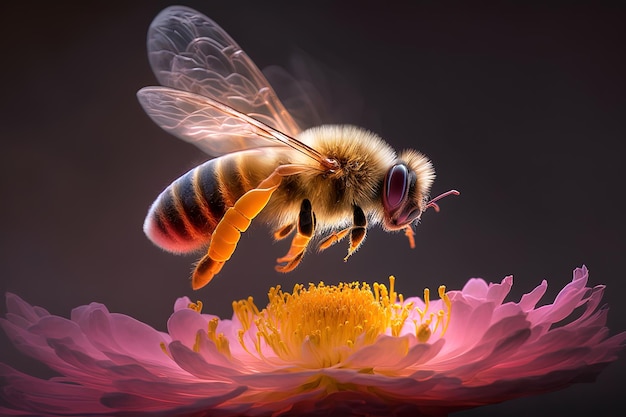This digital illustration captures a detailed and high-resolution image of a bee hovering above a pink flower. The bee, characterized by its soft fur and translucent wings in motion, displays yellow and black stripes on its back, transitioning to a tannish gold around its midsection. Its head, topped with fur resembling a punk rocker’s mohawk, sports two purple antennae and purple eyes. The bee’s legs are yellow and show a build-up of pollen. Intriguingly, a reflection of the flower appears on the bee’s underbelly, giving it a slightly pink hue. The flower, with its long pink petals and a yellow center rich in pollen, is set against a gray background, providing a striking contrast to the vivid subjects.